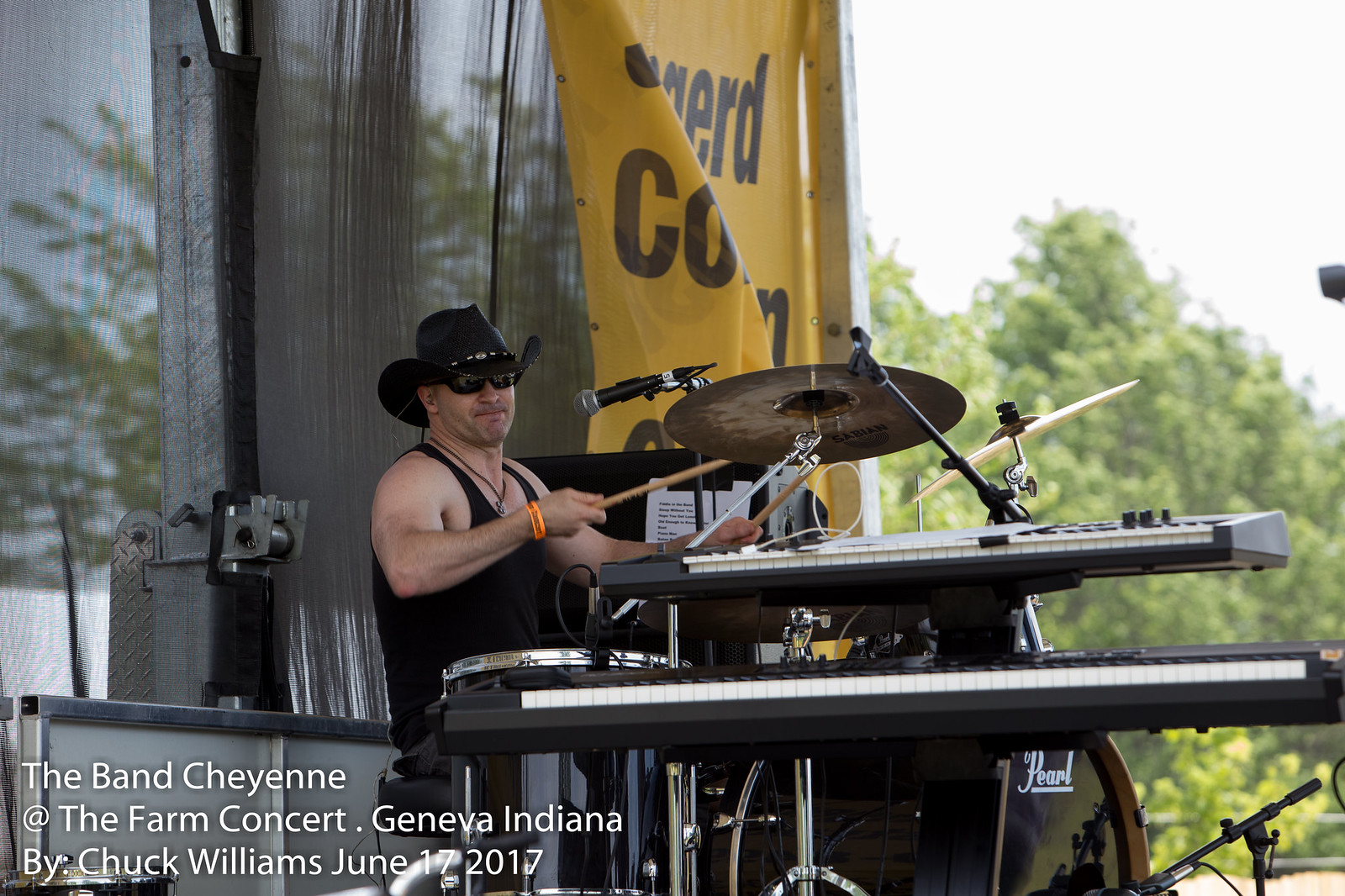In this photograph, labeled in the lower left corner "The Band Cheyenne at the Farm Concert, Geneva, Indiana, by Chuck Williams, June 17, 2017", a drummer is intensely engaged in his performance on an outdoor stage. He is sporting a black tank top, revealing his bare arms and underarms, and a black cowboy hat adorned with silver metal ornaments on the brim. Black sunglasses shield his eyes while an earpod is visible in one ear. Around his neck hangs a black cord with a trinket. His expression is focused, with his mouth tightly closed, his chin drawn down, and his head slightly tilted back as he plays. The drummer's wrists are decorated with a yellow wristband on his left and an orange wristband on his right. Positioned behind a two-tiered keyboard set—with a smaller keyboard on top and a larger one at the bottom—his black drum kit features a cymbal and a bass drum with the emblem "Pearl." A microphone stands in front of him. The backdrop reveals clear daylight skies, some trees, and a yellow banner fluttering in the wind. The presence of curtains adds to the stage setting of this vibrant, open-air concert.